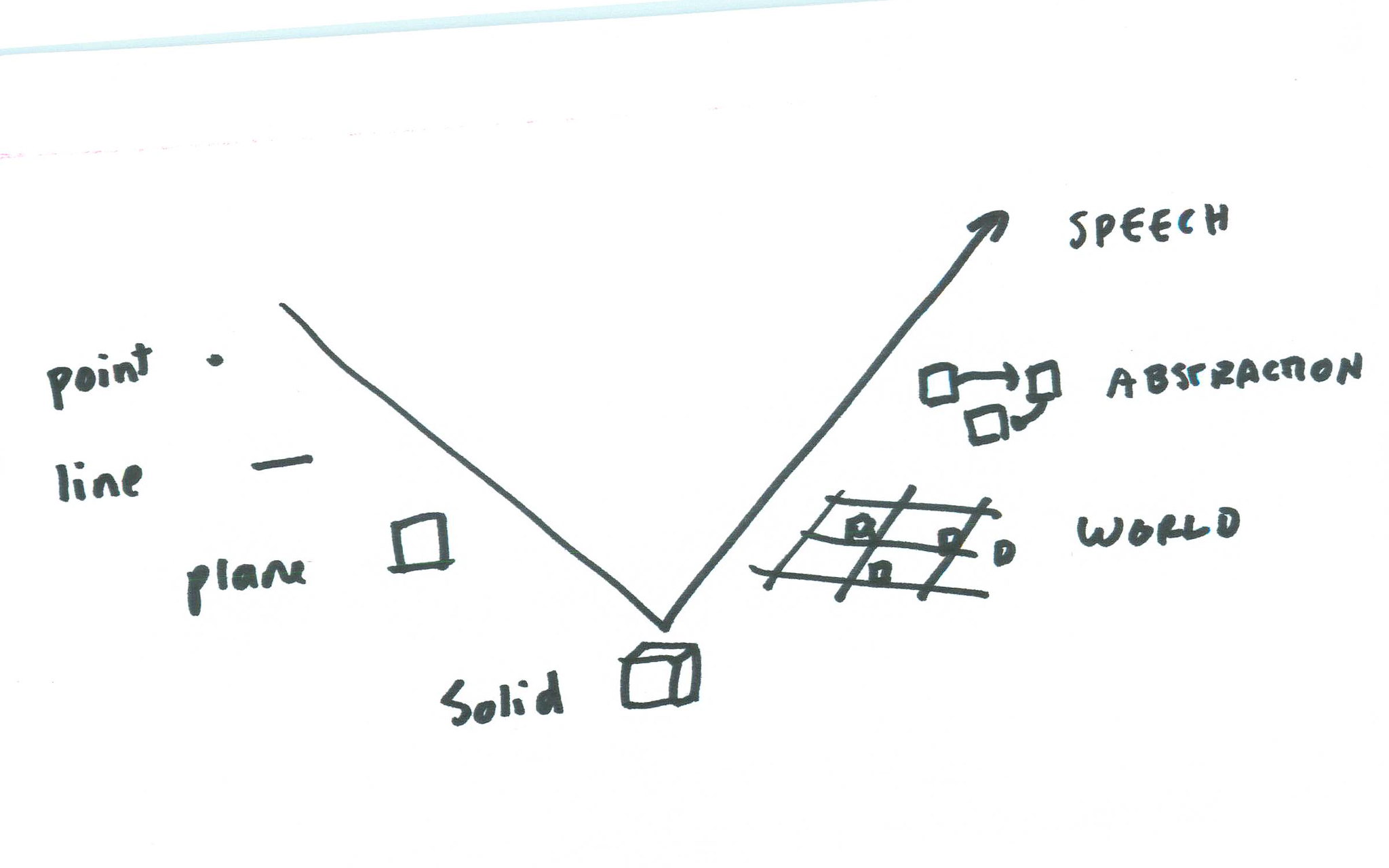This black-and-white drawing features a small, unexpected streak of blue at the very top, which appears to be out of place and unrelated to the artwork. The composition resembles a large 'V' shape—starting from the left, descending downward, and then ascending back up to the right. At the top end of this ascending line, there is an arrow pointing upward.

Along the descending line of the 'V', several key elements are illustrated:

1. At the beginning of the line, the word "point" is inscribed, accompanied by a small dot representing a point.
2. Further down, the word "line" appears next to a simple line illustration.
3. Continuing downward, the drawing features the word "plane" written as "P-L-A-N-E," with a square illustrating the concept of a plane.
4. At the very bottom of the 'V', where the two lines meet, a cube is drawn and labeled "solid."

Transitioning to the upward stroke of the 'V', several more elements are included:

1. Just above the vertex, there is a small tic-tac-toe grid with only four squares, three of which contain star shapes in their corners. This section is labeled "world."
2. Ascending further, three smaller squares are sequentially numbered 1, 2, and 3, with arrows indicating the progression from 1 to 2, and from 2 to 3. This segment is annotated with the word "abstraction."
3. Near the upper end of the right line, the word "speech" is inscribed at the peak.

Each part of the drawing methodically transitions from simple geometry to more complex concepts, culminating in the idea of speech, illustrating a progression from basic elements to higher abstractions.